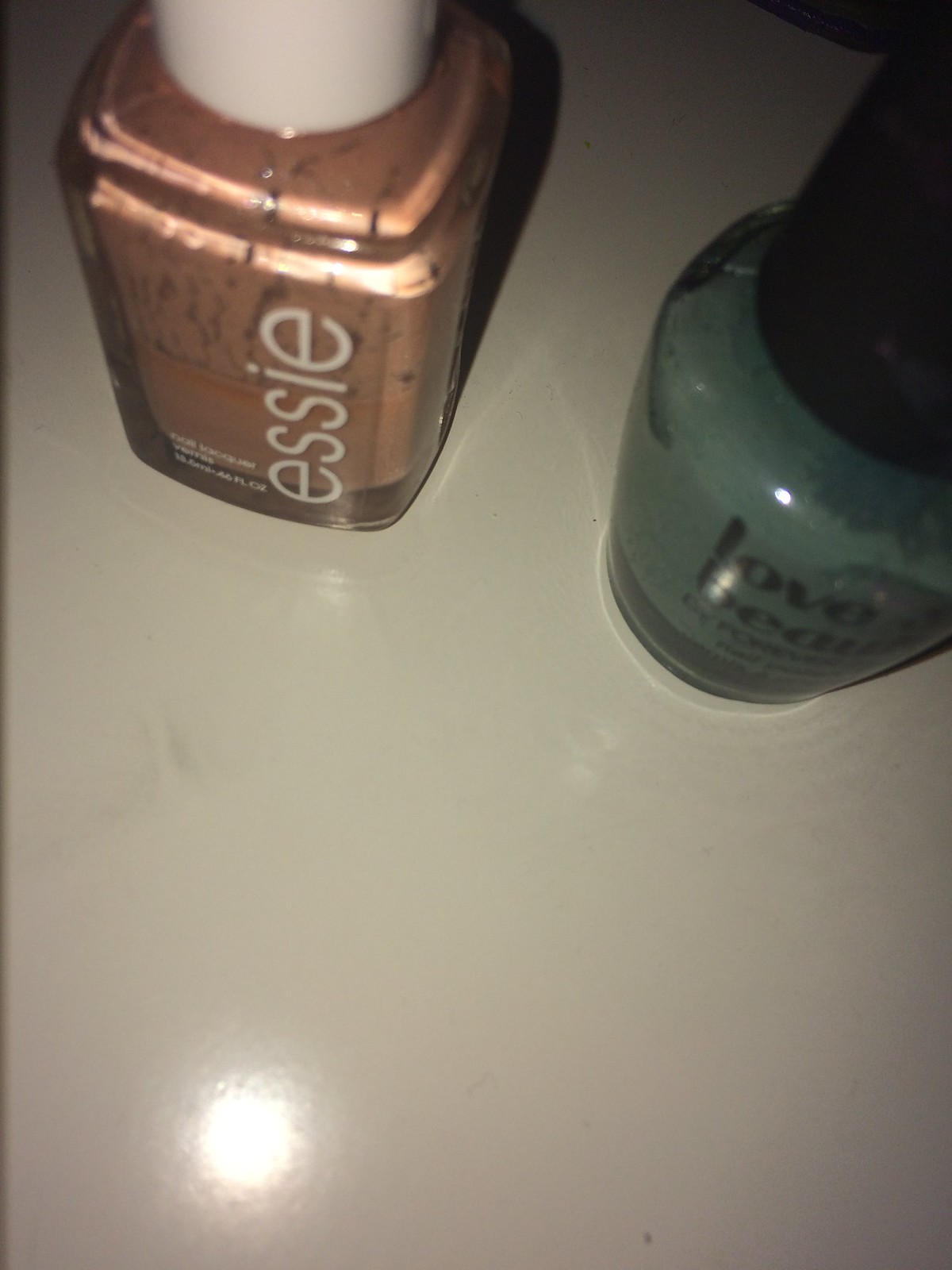The rectangular photograph, taken from a slightly downward angle, captures a pair of nail polish bottles resting on a pristine, shiny white table or desk. In the bottom left corner of the image, there's a noticeable glare from the camera flash. To the left, a half-full bottle of bronze-colored nail polish displays the brand "Essie" in white letters and is topped with a white lid. The bottle on the right, mostly full with a mossy green hue and small speckles of black, has "Love" written on it, partially obscured by "B-E-A-U" underneath, and features a black lid. The clean, bright surface enhances the clarity and detail of the nail polish bottles.